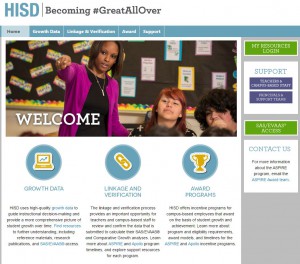This is a screenshot of the "HISD Becoming #GreatAllOver" website, highlighted by a blue banner at the top of the page. The banner includes partially legible navigation options such as "Home" on the left and an indiscernible number of other links, with the last one appearing to say "Support." The overall image is noticeably blurry.

Beneath the banner, there is a "Welcome" image set in a classroom environment, featuring a chalkboard and various vibrant pictures adorning the background. A prominent figure in the scene is a black woman pointing, dressed in a pink jacket, black shirt, and silver necklace. Around her, several high school students are visible, attentively looking towards the direction she is pointing. Notable details include one girl with red hair, another person with black hair, and the indistinct tops of other students' heads.

On the right side of the webpage, there are multiple buttons for user interactions, including "Log In," "Support," "Access," and "Contact Us."

At the bottom of the image, three distinct circles represent different categories: one labeled "Growth Data" with a computer icon, another labeled "Linkage and Verification" featuring chain links, and the final one labeled "Award Programs" depicted with a trophy icon.